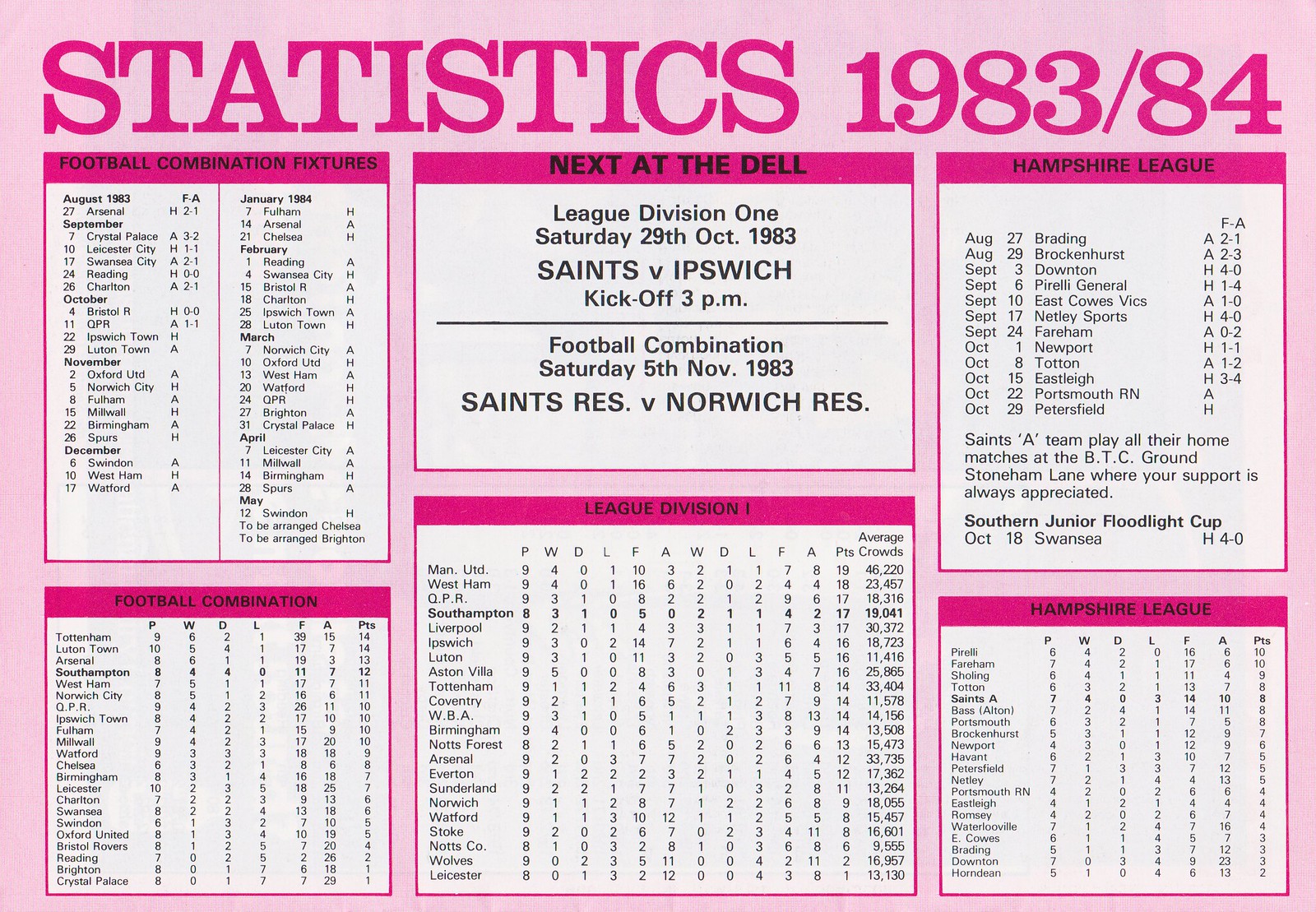In the landscape-oriented image, a light pink and white checkered background hosts a heading in bold fuchsia pink text that reads "Statistics 1983/84." Below the heading, six cards are arranged in two rows and three columns. Each card features a fuchsia bar at the top with black text denoting its title, and a white background below with detailed statistics and schedules in black text. The top left card is titled "Football Combination Fixtures," while the top middle card, deviating slightly, announces "League Division One Saturday 29th October 1983 Saints vs. Ipswich kickoff 3 p.m." beneath a black bar. The top right card is labeled "Hampshire League." In the bottom row, the leftmost card mirrors the top left as "Football Combination," the center card is "League Division One," and the bottom right card, like its counterpart above, is "Hampshire League." Each card is meticulously detailed with dates, match fixtures, and player statistics relevant to the 1983-1984 sports season, catering to avid fans tracking their team’s performance.